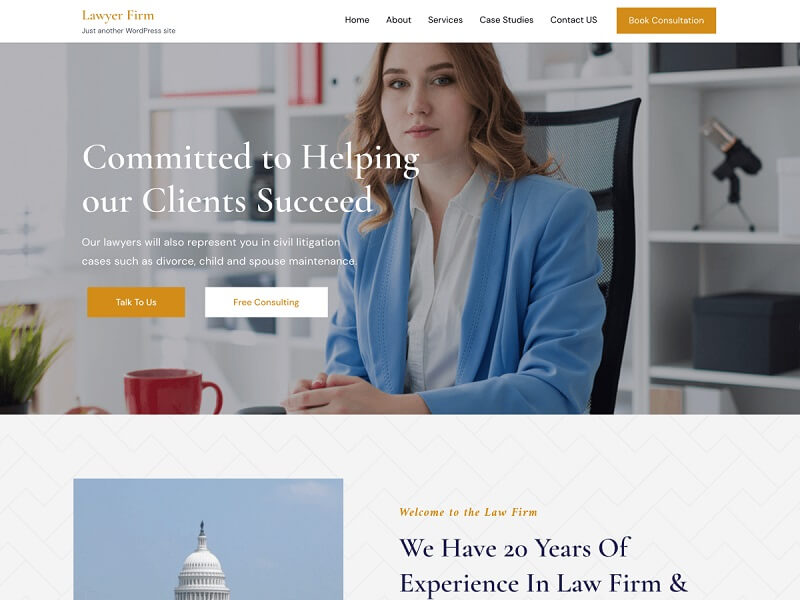Here's a cleaned-up and detailed caption for the described image:

---

The screenshot displays a "Lawyer Firm" website, which appears to be under construction, characterized by placeholder images and text. The top navigation bar includes tabs labeled Home, About, Services, Case Studies, and Contact Us, along with a distinct mustard yellow "Book Consultation" button. Dominating the page is a banner area with the headline "Committed to Helping Our Clients Succeed." The banner features an image of a white woman sitting at a desk in an open, pristine, white-colored office. On the desk sits a red mug, and the background features shelves, some containing various items including what appears to be a small, possibly telescope-like device likely intended for web conferencing.

Below the banner section, there's a segment that begins with a statement, "We have 20 years of experience in the law firm," accompanied by an image of the U.S. Capitol building's dome. Additional text, "Our lawyers will also represent you in civil litigation cases such as divorce, child and spouse maintenance," is present along with two call-to-action buttons labeled "Contact Us" and "Free Consulting."

The website layout suggests it belongs to a professional legal firm dedicated to extensive client support and expertise in various areas of law.

---